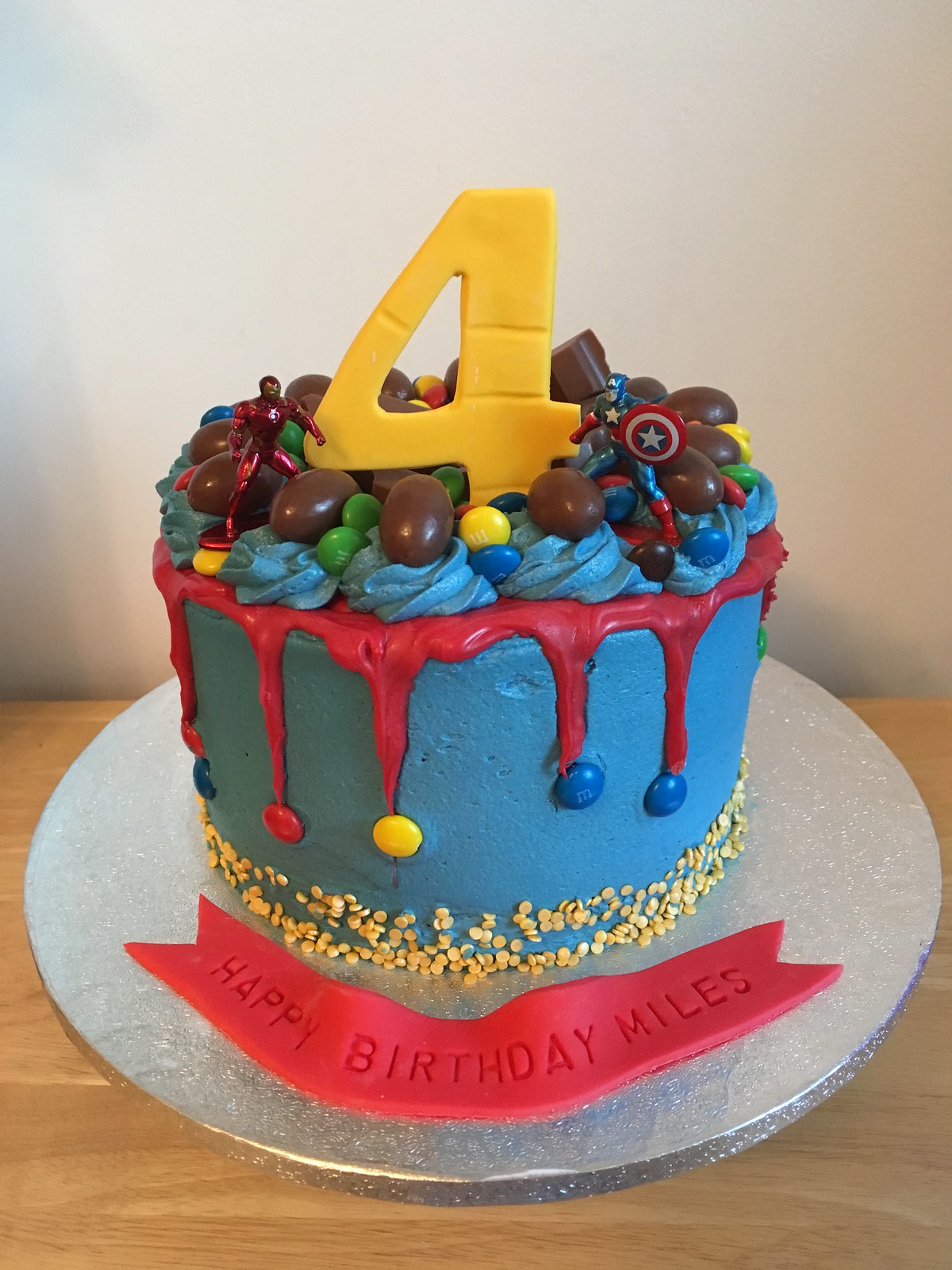In the photograph, a blue birthday cake stands prominently on a silver glittery platter, set atop a brown wooden table. The cake features vibrant blue icing and is adorned with an array of colorful decorations. At the base, small yellow candies encircle the cake, and red icing appears to drip artfully down the sides. Each drip is punctuated by an M&M at the bottom. A red icing banner, likely made of sugar or frosting, spans the front of the platter, bearing the message "Happy Birthday Miles."

The top of the cake is a celebration of colors and textures, featuring multiple colored M&M's and blue swirls intricately designed with chocolate eggs perched on top. A large yellow number 4, likely crafted from sugar or frosting, stands upright as the central decorative element. Additionally, two small action figures, including one resembling a superhero with a shield marked by a star, embellish the cake, adding a playful touch to the design.

The overall composition is rich and detailed, highlighting the cake's multi-layered, whimsical decor. Both the platter, possibly covered in aluminum foil to create its glittery effect, and the wooden table contribute to the festive ambiance, with a white wall serving as a neutral backdrop.